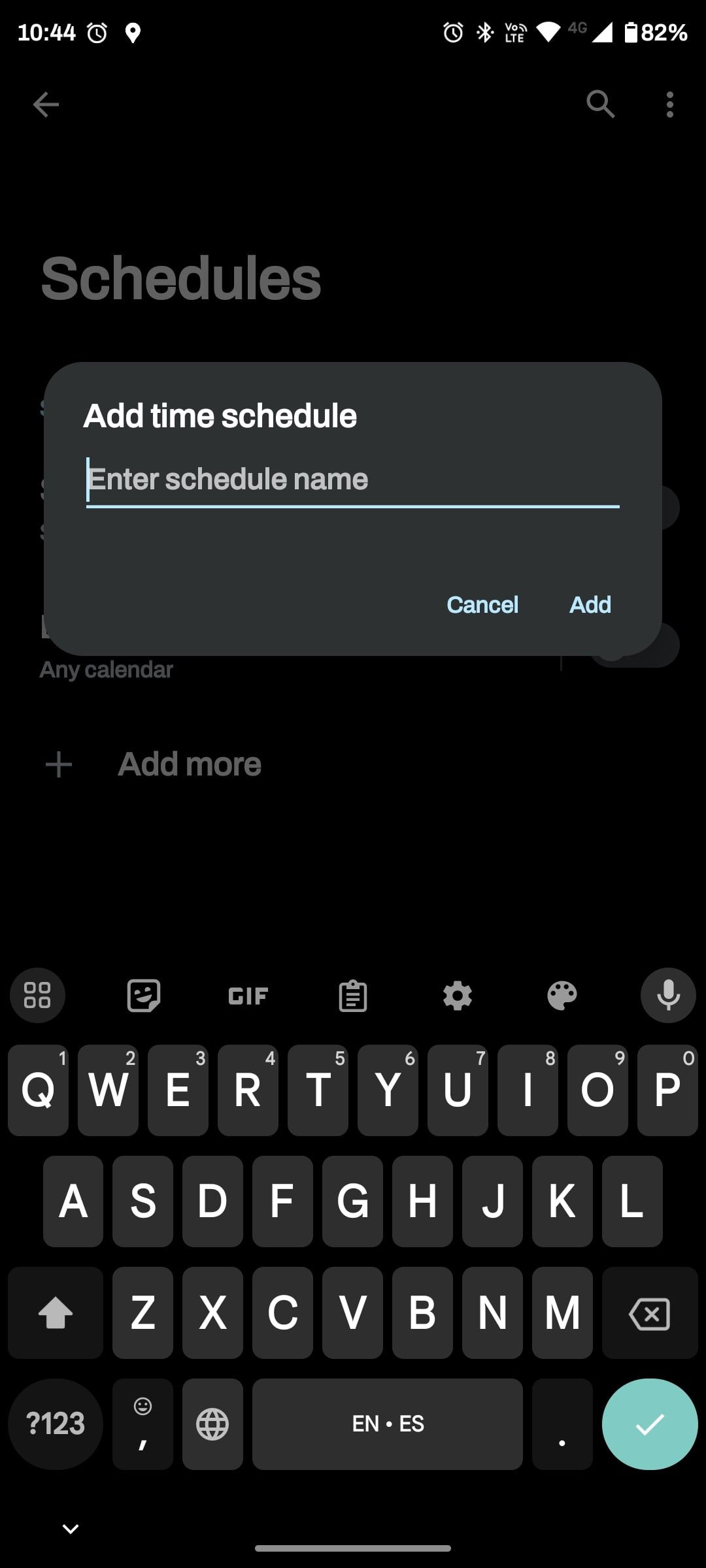The image depicts a screenshot of a smartphone screen. In the top left corner, the time is shown as 10:44, accompanied by some small icons. To the right, the full bars of the Wi-Fi icon indicate a strong connection, and the battery icon shows an 82% charge. All these elements are set against a black background with light gray text.

Below the status bar, the screen displays the word "Schedules." A bordered section below this prompts the user to "Add time schedule," with a cursor blinking next to the instruction "Enter schedule name." Light blue "Cancel" and "Add" buttons appear below this entry field.

Further down, an "Add more" bar is visible, followed by more black space that includes icons to add a GIF, access settings, select colors via an artist palette icon, and use a microphone. The QWERTY keyboard is displayed against a dark background, with white keys. In the bottom right corner, a blue circle with a white check mark stands out.